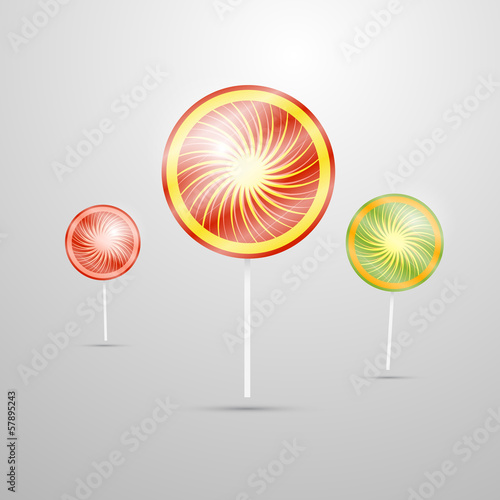This stock photo features a trio of swirled, circular shapes resembling lollipops set against a gradient background that transitions from gray to white, moving diagonally upwards to the right. The lollipops are mounted on white sticks. 

The central lollipop is the largest, adorned with an outer red ring, a yellow circular border, and a yellow sunburst at the center, evoking the image of the sun. 

To the left, the smaller lollipop has a layered design, starting with an outer red ring, followed by a pink ring, and culminating in a red sunburst at the core with a lighter pink center, creating a gradient effect. 

The lollipop on the right is green with a yellow sunburst at its center, encircled by a gold-yellow ring and finished with an outer green ring, completing the vibrant and whimsical visual composition.